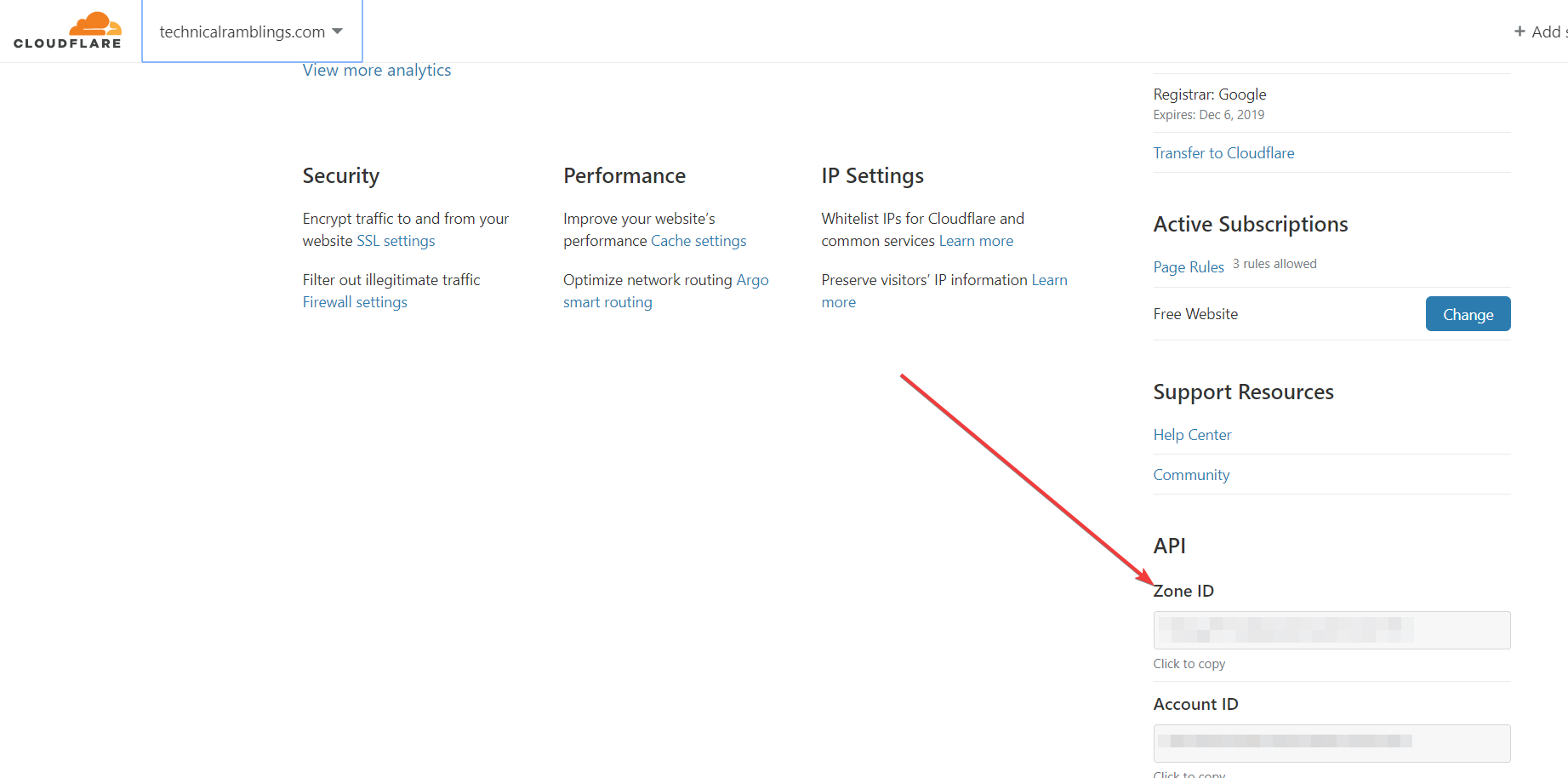This is an annotated screenshot from the CloudFlare dashboard. In the top left corner, the CloudFlare logo is displayed in all black capital letters: C-L-O-U-D-F-L-A-R-E, with an orange cloud icon positioned above the part of the name that says "Flare." To the right of the logo, "TechnicalRamblings.com" is listed as the domain. Below this, there is an option labeled "View More Analytics."

The main body of the screenshot has a white background and is segmented into various sections with headings and descriptions. Under the section titled "Security," it mentions features like "Encrypt traffic to and from your website" under SSL settings and "Filter out illegitimate traffic" under firewall settings.

In the "Performance" section, features are described such as "Improve your website's performance" with cache settings and "Optimize network routing" with Argo Smart Routing. 

In the section related to "IP Settings," it provides options to "Whitelist IPs for CloudFlare and Common Services" with a link to "learn more" and "Preserve visitor's IP information" with another "learn more" link. 

The "Registrar" section details that the domain is registered with Google and will expire on December 6th, 2019, with an option to "Transfer to CloudFlare."

Under "Active Subscriptions," it mentions "Page Rules," allowing three rules on a free website, with an option to "Change."

The "Support Resources" section provides links to the Help Center and Community forums. 

In the "API" section, there is a "Zone ID" with a red arrow pointing to the word "zone." Although the field has been filled out, it is blurred for privacy, and there is an option to "Click to copy." Similarly, the "Account ID" field is also blurred, with the same "Click to copy" option below it.